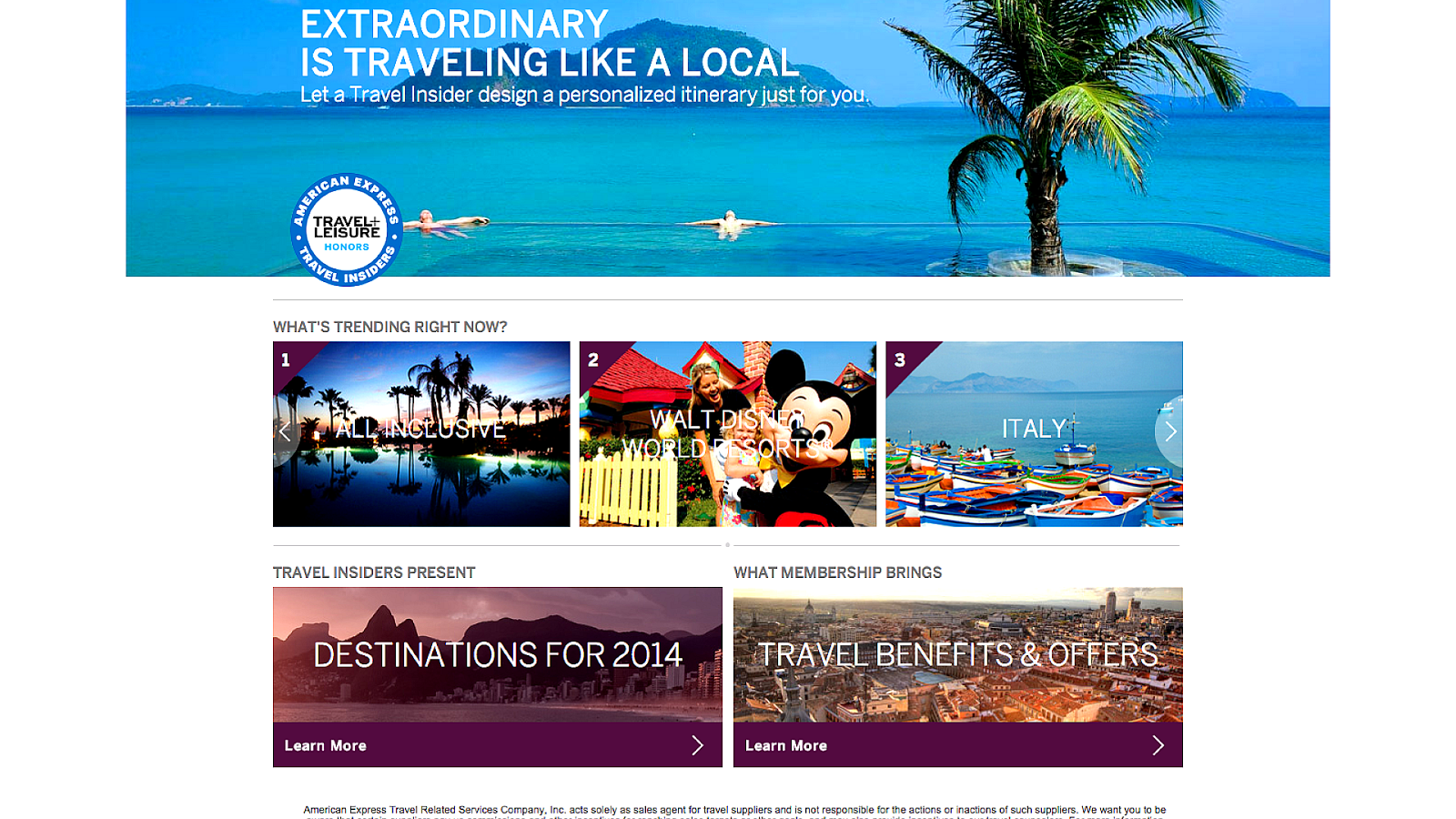This image appears to be a vibrant promotional graphic related to travel, specifically highlighting a variety of travel destinations and a rewards program. The central text in bold white reads, “Extraordinary is Traveling Like a Loco,” suggesting an exhilarating and unconventional travel experience. The background features stunning visuals including a serene beach scene with a palm tree, reminiscent of a tropical paradise.

Additional text reads, “What’s Trending Right Now: Travel Insiders Present What Membership Brings.” This implies the graphic is advertising the benefits of a travel membership program. There's a prominent blue circle bearing the text “American Express Travel Insiders” and “Travel + Leisure Honors,” indicating that this could be part of a premium travel rewards program offered by American Express.

The image includes snapshots of various destinations such as a lively Walt Disney Resort with a cheerful Mickey Mouse, picturesque scenes of Italy featuring boats, and the urban splendor of a bustling city—likely New York. Different captions such as "Travel Benefits" and "All-Inclusive Destinations for 2014" emphasize the diverse travel experiences available through this program. An arrow on the right suggests interactive elements, possibly for browsing more destinations or offers.

In summary, this appears to be a comprehensive advertisement for a travel rewards program showcasing enchanting travel opportunities like exotic beaches, iconic theme parks, and cultural hubs, all designed to entice prospective travelers to join the membership and explore the world.